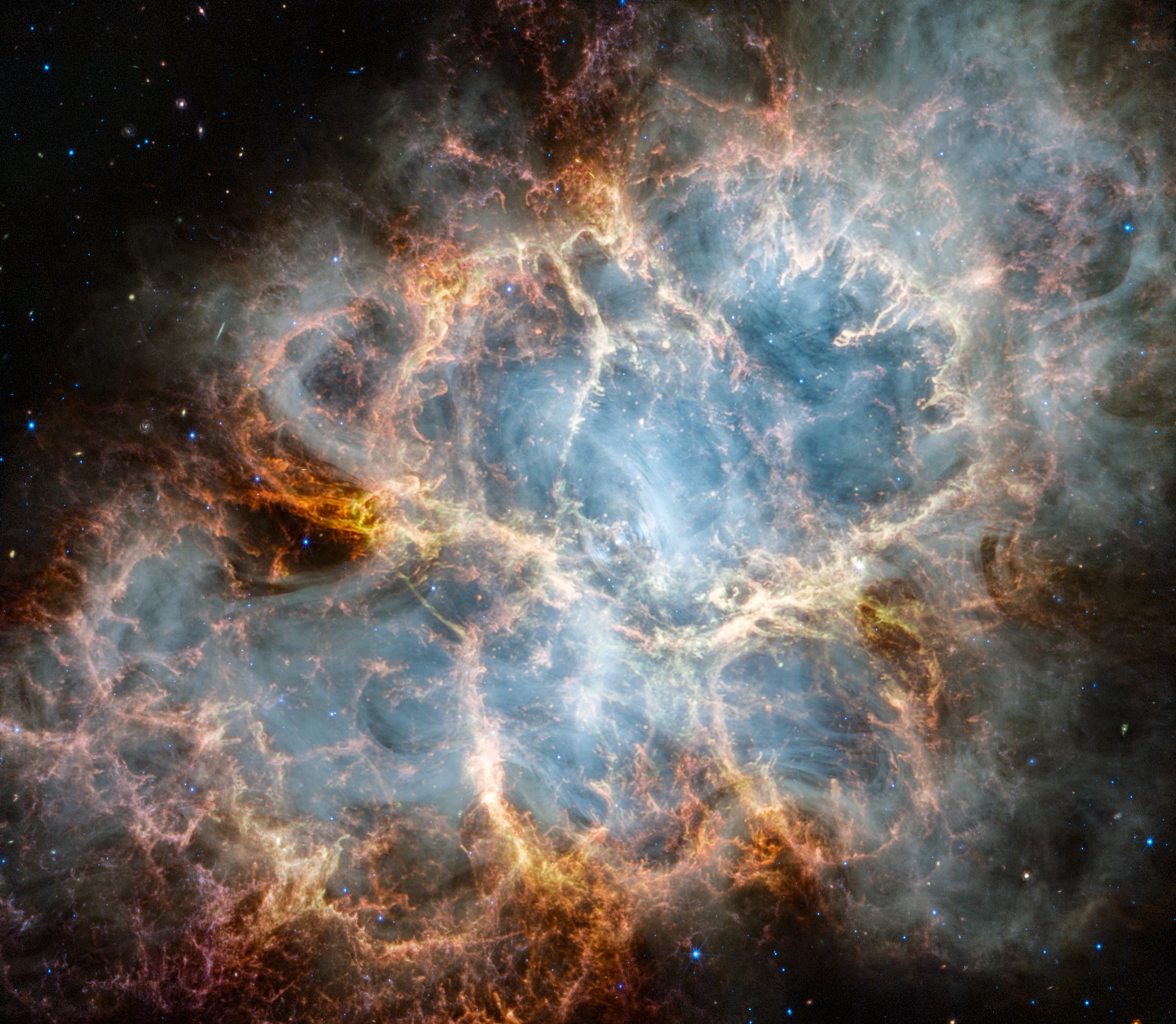This image captures the ethereal beauty of the Crab Nebula, as envisioned by a space telescope. Dominating the scene is a vast, cloud-like formation extending from the upper right to the lower left, encompassing a variety of intricate details. The core of this nebulous mass is primarily blue, giving way to wisps of white that mimic lightning strikes or veins, and are highlighted by patches of dark gray and brown. Surrounding the nebula, the peripheries flaunt a rich medium to dark brown hue, resembling molten lava. The black expanse of space envelopes this vibrant spectacle in the upper left and lower right corners, dotted with sparkling white, blue, and red-tinged stars. This celestial marvel, with its smoky, dense golden areas and an almost coral-like formation in the lower left, presents a dramatic and mesmerizing view, blurring the line between reality and fantasy.